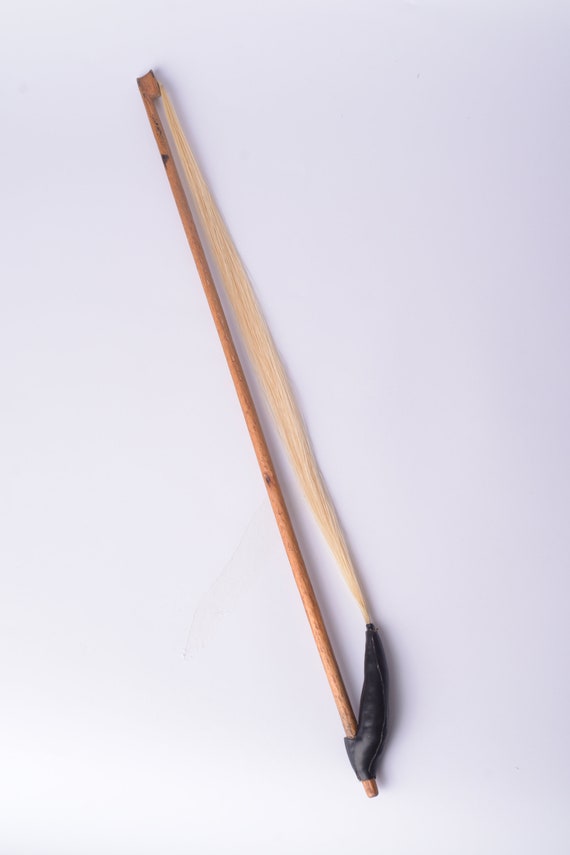The image features a handmade object that closely resembles a rudimentary slingshot or bow, crafted from a wooden stick. The wooden piece, which has a circular cross-section and is brown in color, extends diagonally across the image, nearly filling the frame. It rests on a background that appears to be a muted purple or light blue, though some described it as white. Attached to the wooden stick is a black leather or electrical tape band, wrapped around the bottom end, creating a makeshift handle. Extending from this handle is a string or yarn-like material that stretches up to the opposite end of the stick. The string appears to be secured with the same black tape. This contraption, seemingly made from found materials, lacks any formal labeling or descriptions in the image, enhancing its appearance as a homemade, improvised tool or toy.